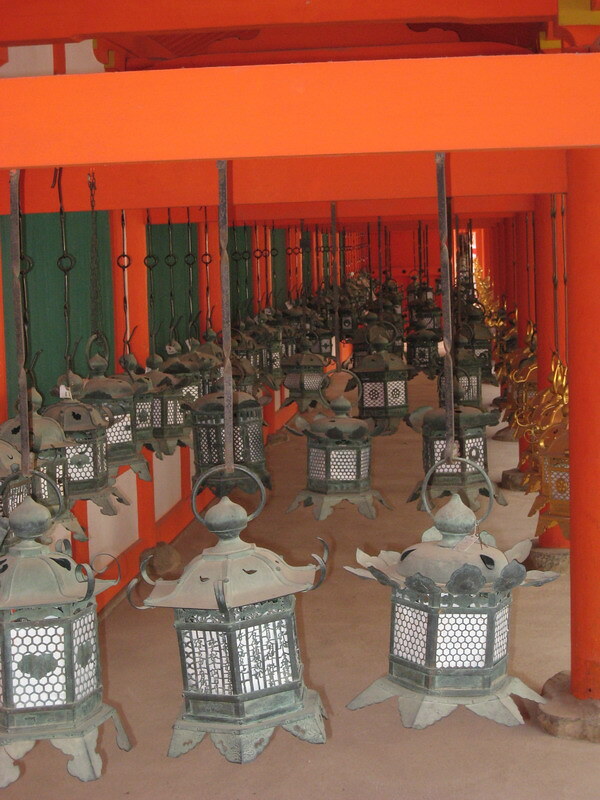The image depicts a small, elongated hall adorned with numerous ornate Chinese lanterns. This hall's striking interior features red-painted walls, ceilings, beams, and circular columns supporting the beams, creating a rich, vibrant setting. The lanterns, which appear quite dusty, are made of iron and feature hexagonal (octagonal) shapes framed by decorative metal bases reminiscent of petals. They are suspended from the ceiling by metal hooks, enhancing the room's traditional ambiance. Additionally, there are hints of green elements—possibly closed windows or doors—on one side, along with white panels interspersed among the predominantly orange backdrop, giving the room a unique, layered aesthetic. The lanterns range in color, with some looking gold while others appear silver and gray, emphasizing the hall’s mix of vintage and cultural charm.